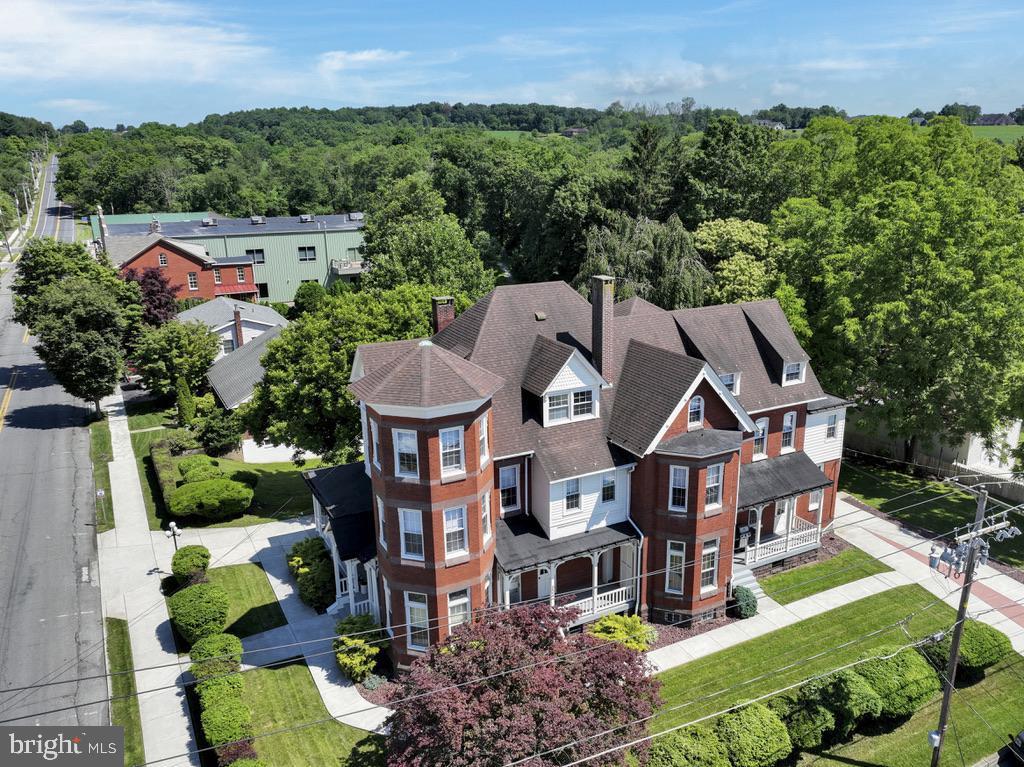This image is an overhead aerial shot of a stunning Victorian-style mansion situated on a well-manicured corner lot. The house, which features both red brick and white siding, boasts a three-story structure complete with several dormers, a charming turret on the left, and a grand wraparound porch with elegant white railings supported by columns. The roof, covered in brown shingles, crowns this architectural gem. The manicured lawn is adorned with neatly trimmed hedges, vibrant green bushes, and a distinctive tree with purple leaves. A cement walkway elegantly curves through the property, leading to neatly kept driveways on either side of the house. Surrounded by mature green trees, the mansion stands out amidst a picturesque backdrop, which includes a blue sky and distant mountains. Power lines are noticeably present, running over the front yard and adding an element of everyday urban life. Behind the house, additional residential buildings can be seen, though the main focus remains on this luxurious property. The lower right corner of the image features the branding of Bright MLS, highlighting its listing status.